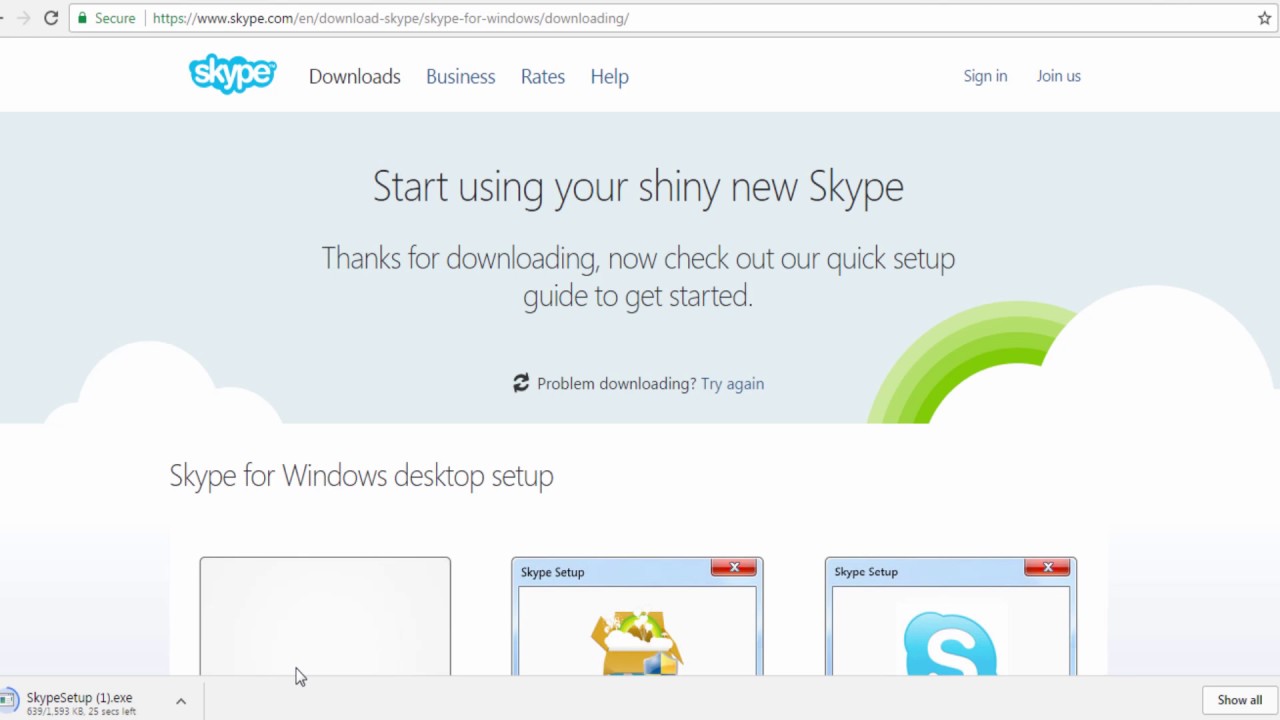The screenshot displays a browser window showcasing the Skype download webpage. The browser's layout is wider than it is tall and features a thin gray banner at the top, which is partially cropped on the left. This banner includes standard browser navigation buttons such as forward, back, and reload.

Below the gray banner, there is a white address bar displaying the secure URL, which is a lengthy English link pointing to a Skype.com page for downloading Skype. 

Under the address bar is another white banner featuring the familiar blue Skype logo on the left. Next to the logo are navigation options labeled "Download," "Business," "Rates," and "Help." Towards the right side of this banner, there are options to "Sign In" and "Join Us."

The main content area beneath this banner includes a graphic dominated by blue hues with some cloud imagery at the bottom and a multicolored, green-tinted rainbow. Text within this graphic reads "Start using your shiny new Skype." Below this, instructions say "Thanks for downloading. Now check out our quick setup guide to get started," followed by a smaller text link: "Problems downloading? Try again," which is clickable and colored blue.

Near the bottom, the webpage highlights the "Skype for Windows Desktop" setup process with three different images, though the tops of these images are cut off.

At the very bottom of the screenshot, a gray download banner displays "SkypeSetup1.exe," indicating the downloadable file, with a "Show All" button on the far right.